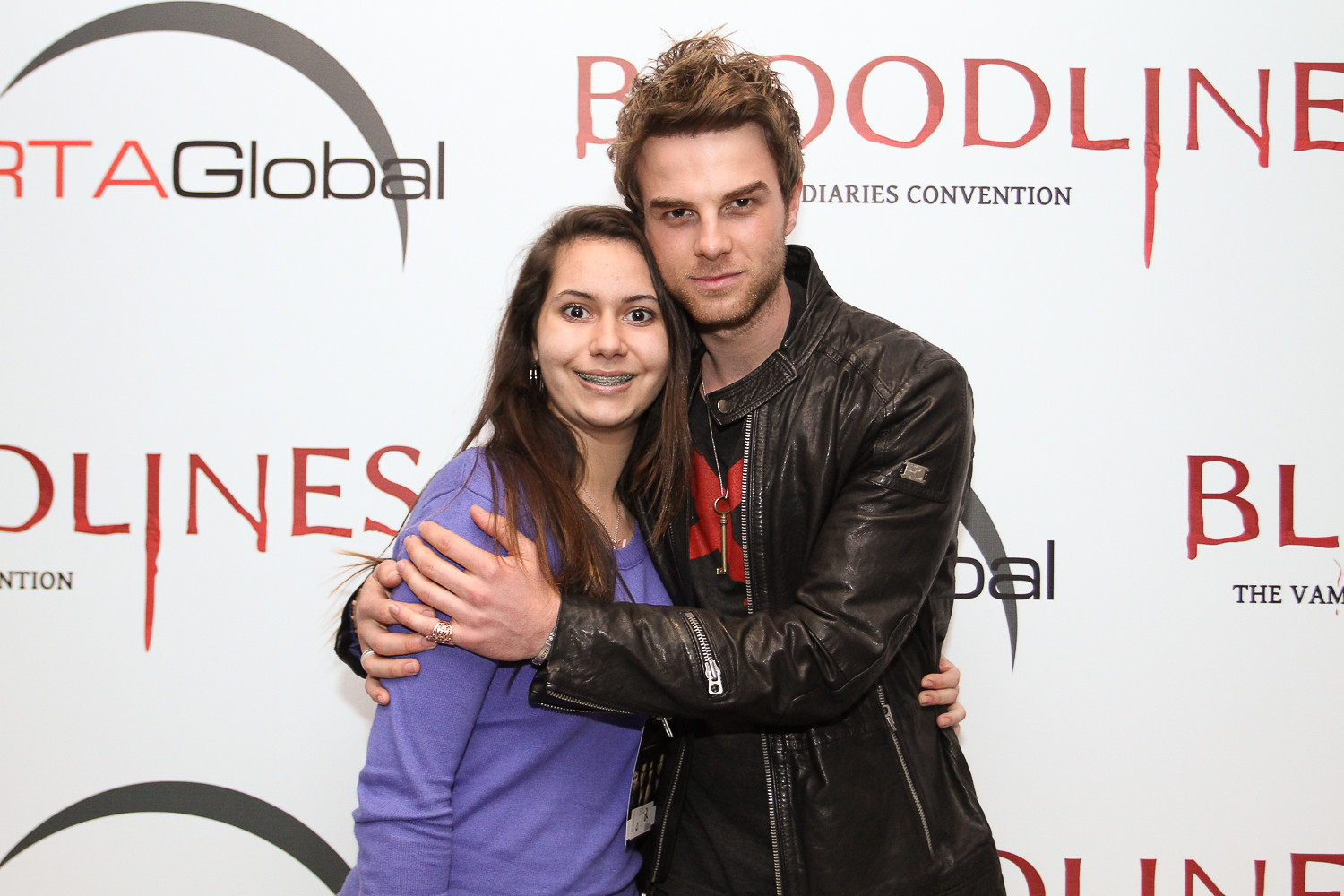The image depicts a man and a woman standing in front of a white backdrop, typical of a red carpet or convention setting. The backdrop has "Bloodline" written in red, with the text appearing to drip like blood, and "The Vampire Diaries Convention" underneath. There is also a logo for RTA Global visible among the fragmented and partially cut-off sponsor names. The man, who has short, blondish hair with dark roots, is wearing a black leather jacket over a black and red shirt, and he has rings on both his pinky and ring fingers of his right hand. He is embracing a young woman with long dark hair, dark eyes, and is wearing a purple sweater or sweatshirt. The woman, who appears to be a fan, is smiling and looks ecstatic yet nervous. She also has braces and is wearing earrings, along with a lanyard around her neck. The overall impression is that they are at a fan event or movie premiere related to The Vampire Diaries.